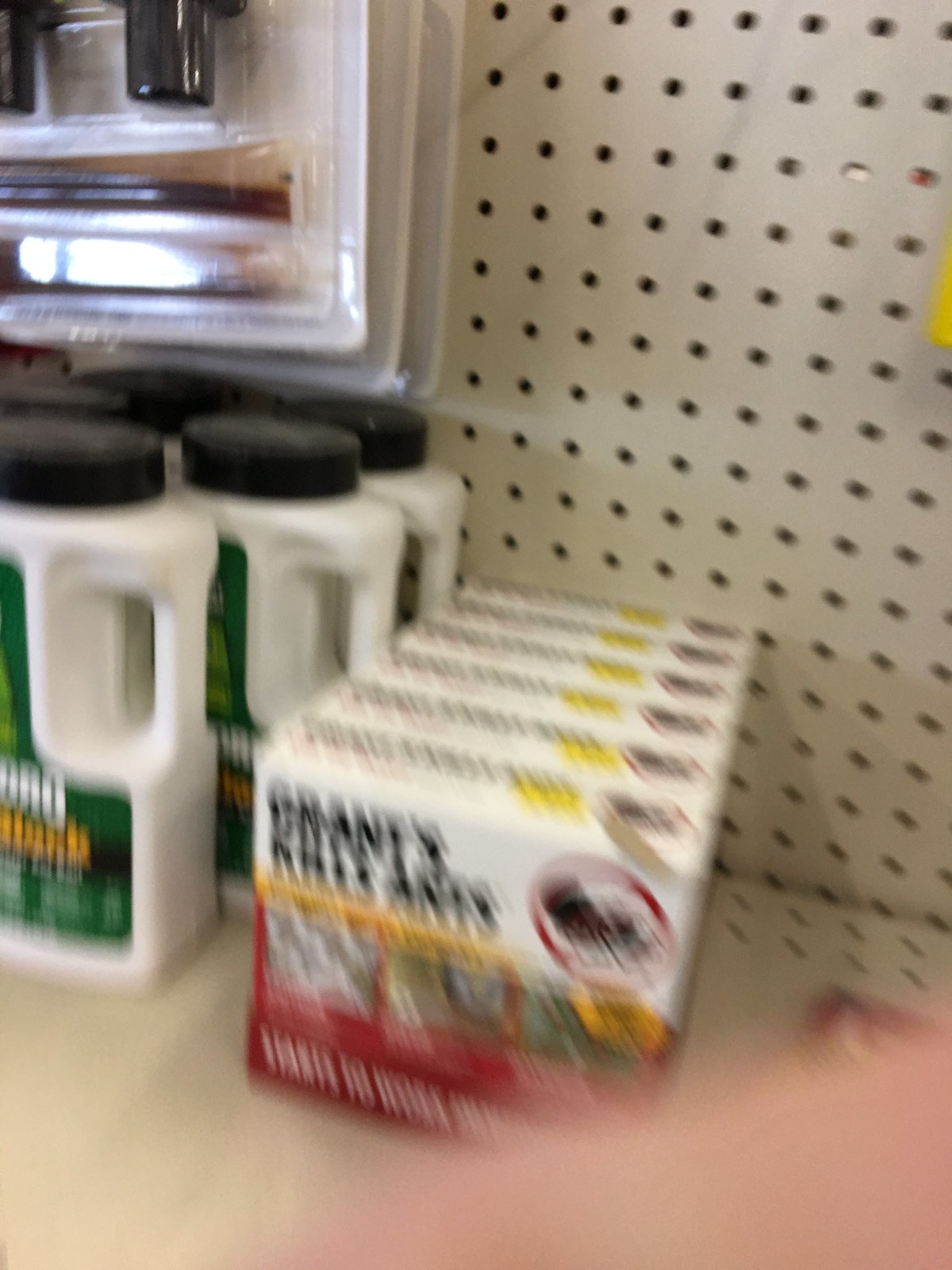This photo, taken in portrait orientation with a cell phone camera inside a store, is quite blurry, particularly towards the bottom. A finger partially obscures the lens from the bottom right to the center, contributing to the image's poor quality. The clearest part of the image is near the top, where six identical boxes are stacked in a row, with only the front face of one fully visible. The boxes display a white border with some yellow and a red bottom border. The label reads "Grant's Kills Ants" in black letters on the white border and features a picture of what seems to be an ant in a red circle. Below the text, there is a yellow border with several indistinguishable images due to blurriness. On the left-hand side of the photo, a white container with a black round cap and green labeling, potentially another pest control product, can also be seen.